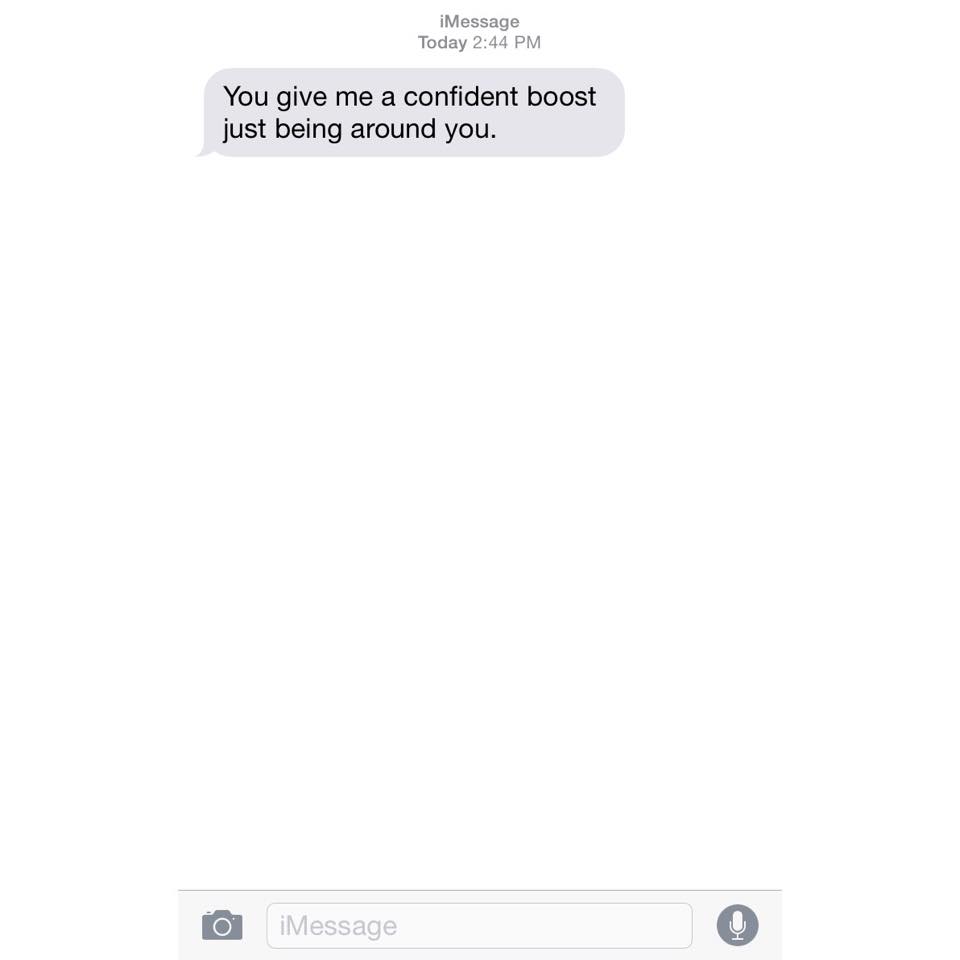A screenshot from an iPhone's iMessage app is displayed, capturing a conversation timestamped "Today, 2:44 PM." The screen shows a heartfelt message sent to someone, where the sender praises the recipient for their positive influence, saying, "you give me a confident boost just being around you." Notably, the sender used the word "confident" instead of the more grammatically correct "confidence." The chat thread is devoid of any other messages or responses, highlighting the solitary nature of this affectionate statement. At the bottom of the screen, there is a text entry box labeled "iMessage," flanked by a camera icon on the left, intended for sending photos, and a microphone icon on the right, likely for voice recordings. The minimalist interface and the absence of additional content emphasize the simplicity and sincerity of the message conveyed.